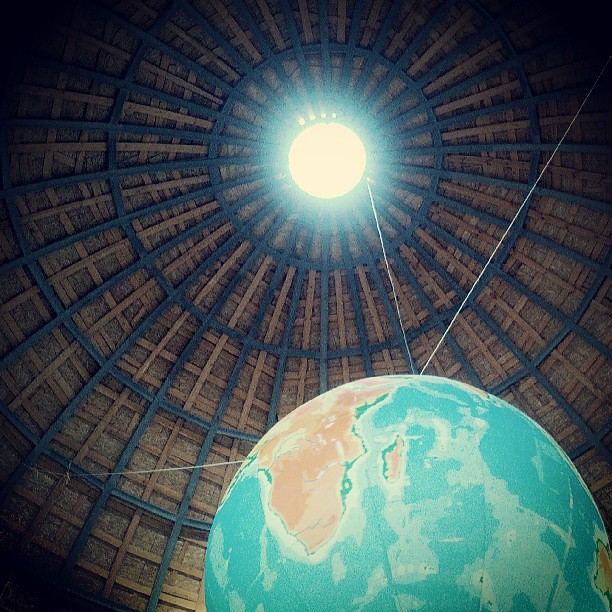The image captures the interior of a unique, dome-shaped hut constructed from alternating layers of black and brown plywood. The dome's intricate woodwork spirals downwards, creating a mesmerizing pattern that culminates in a round opening at the top, allowing light to stream in. Suspended beneath this opening is a large, detailed globe of Earth, prominently featuring Africa, the surrounding ocean, and parts of other continents. The globe, colored in shades of blue and tan, is held up by numerous white ropes that converge at a single white string, securing it to the ceiling. The natural light filtering through the circular aperture bathes the globe in a soft, yellow-white glow, highlighting its features and emphasizing its suspended position within the captivating wooden structure.